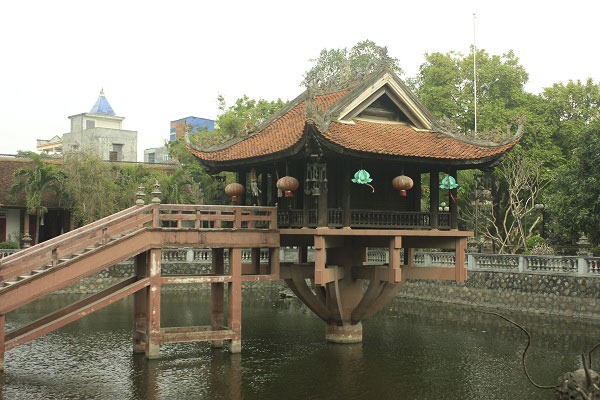This landscape photograph captures a serene, Asian-inspired scene centered around a pagoda built atop a single post within a man-made pond. The pagoda, showcasing a blend of Chinese architecture and hints of French Indonesian influence, features a triangular shingled roof with upturned corners, characteristic of traditional Chinese design. Colorful brown and green lanterns dangle from its eaves, adding a vibrant touch to the tan wooden structure. A dock extends diagonally from the pagoda towards the lower left corner of the image, transitioning into wooden stairs that descend into the water. A stone seawall with a fence borders the pond, leading into a lush park area filled with verdant trees. In the background, beyond the greenery, a row of tan and yellow buildings with blue roofs stands under a white sky, completing this tranquil outdoor daytime scene.